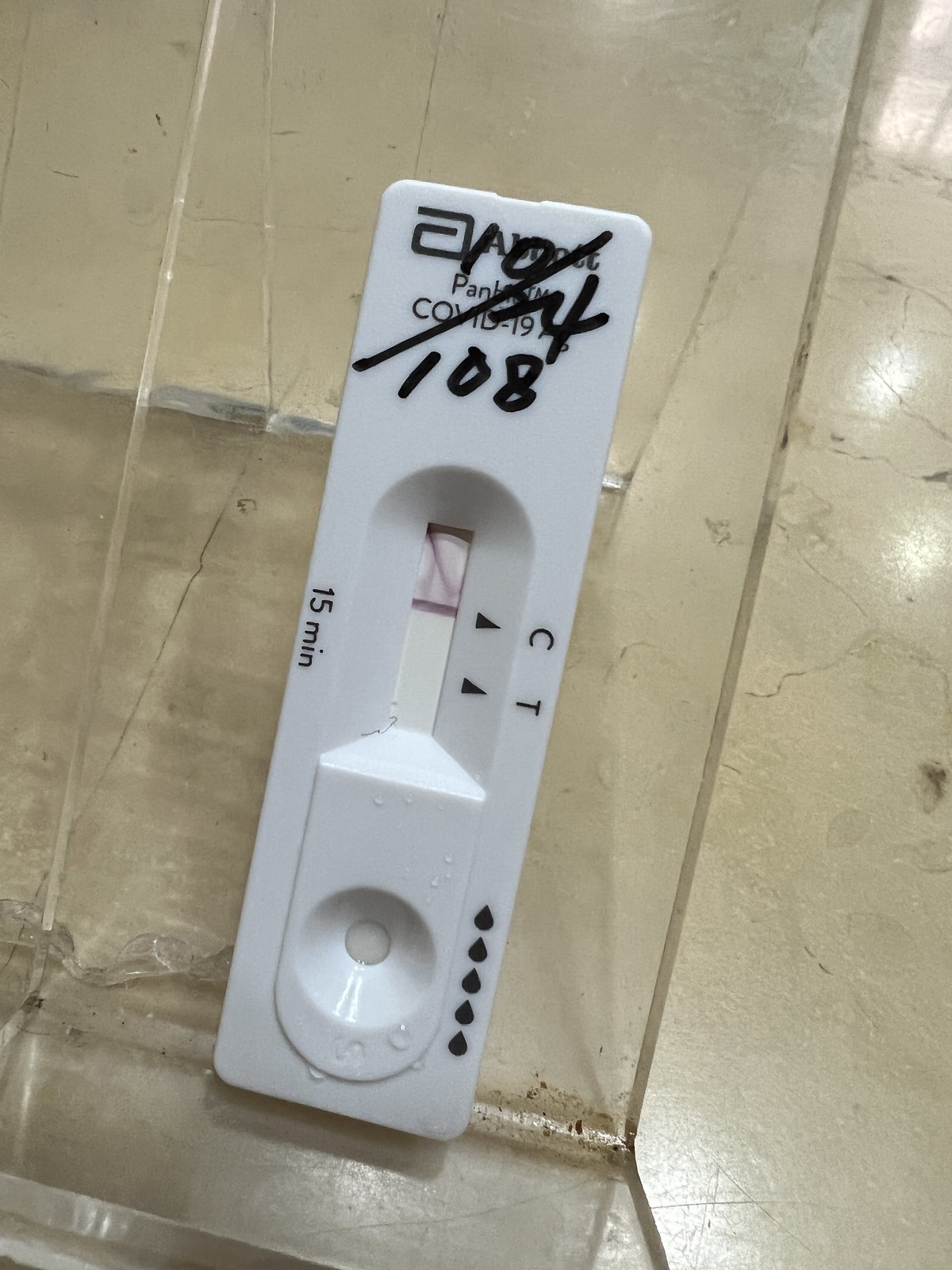This color photograph prominently features a COVID-19 rapid antigen test kit positioned in the center of the frame. The kit is placed on a light grayish tile surface, which is illuminated by bright light reflecting from the upper right side. At the very top of the test kit, the pre-printed label "COVID-19" is visible, though partially obscured by handwritten notations in black magic marker. These notations include a series of numbers: a slash line, the number 4, and the number 108.

The test kit itself is white and oblong in shape, with various details marked on its surface. Below the handwritten notes, an indentation indicates the test area. Along the side, the label "15 MIN" specifies the test duration. Near the upper section of the kit, the letters "CT" can be seen, likely denoting control and test lines. At the bottom part of the test, another indentation is present. On the right side of this indentation, there are five black teardrop-shaped dots, arranged vertically.